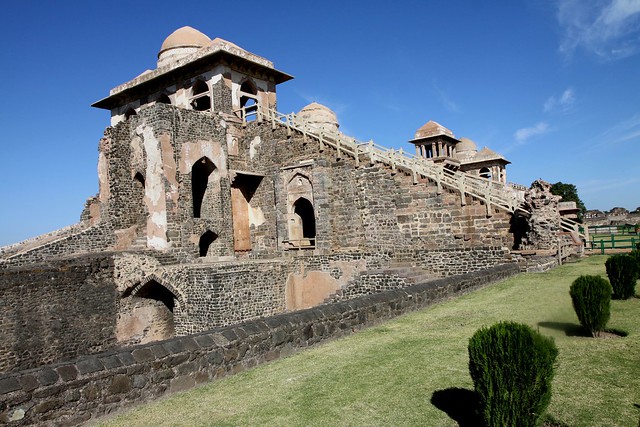This horizontally aligned rectangular photograph captures an ancient, weathered stone structure under a blue sky with a few feathery clouds in the upper right corner. The main subject is a large, light and medium brown brick construction that stretches diagonally across the middle of the image. This structure appears to have multiple cutouts and archways, which suggest entry points. The top of the structure features small domed tops and railings, indicating it may serve as a viewing area. The lower portion includes a low-level retaining wall. 

Toward the right side of the image, there is a grassy knoll adorned with darker green bushes, neatly spaced apart. Further in the background, other distant structures and possibly picket fences are faintly visible. This historic building, characterized by its weathered appearance, includes a long brick stairway that connects to another similar brick structure. A ramp also seems to provide access to the top. Despite being ancient and evidently subjected to preservation efforts, the structure stands robustly, seemingly raised above a moat or similar surrounding feature. The overall scene blends elements of resilience and decay, encapsulated in a picturesque, possibly European, setting.